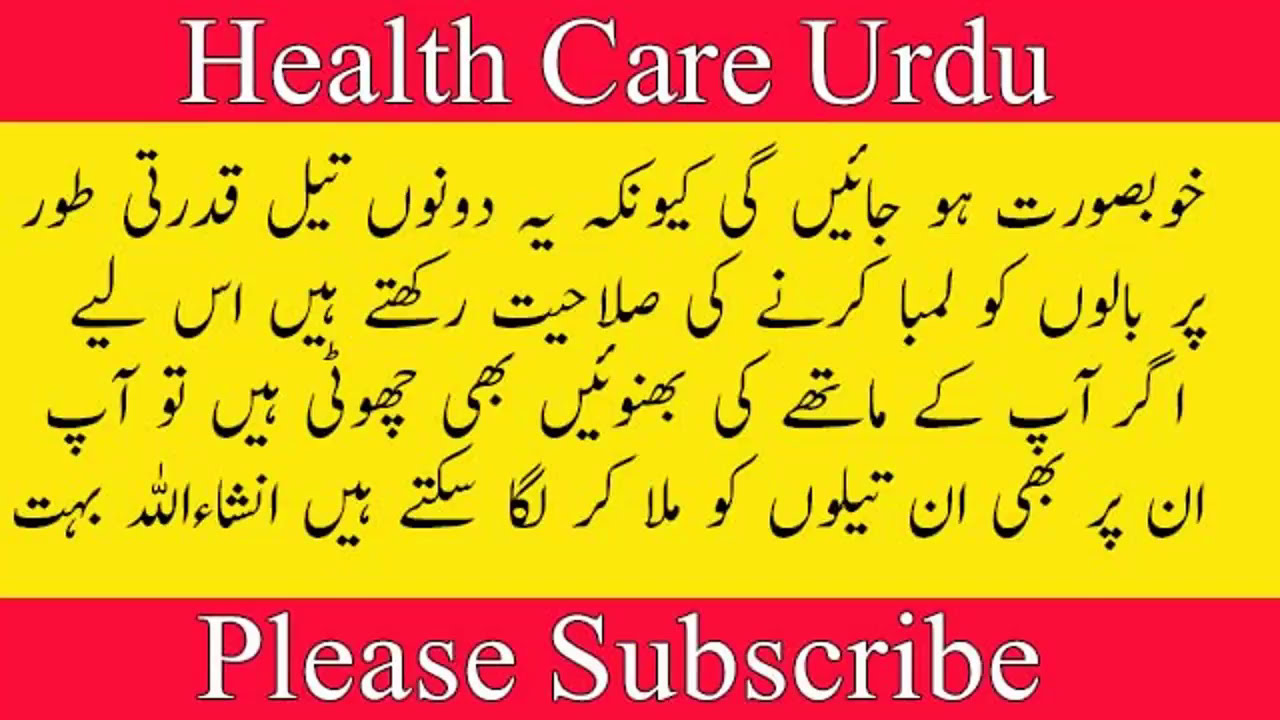The image is divided into three horizontal strips, resembling a flag. The top strip is a small red bar featuring bold white text that reads "Health Care Urdu." The middle, larger strip is yellow with four lines of black Urdu text. The bottom strip is again red, similarly bearing bold white text that says "Please Subscribe." The Urdu letters in the yellow section are clearly visible in black, and the formatting of the white text uses capital letters for emphasis: H, C, U in "Health Care Urdu" and P, S in "Please Subscribe." This design suggests an advertisement or informational banner likely related to healthcare.